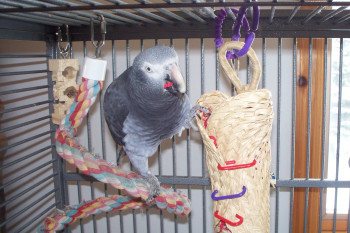The photograph depicts a well-lit indoor scene focusing on an intricately detailed gray metal birdcage with thin blue bars. The birdcage is open at the front, offering a clear view inside, where a striking parrot perches. The parrot, primarily dark gray with a gradual fade into lighter gray and white hues, features a white face and a distinctive beak that is white on top and black on the bottom. Its beady black eyes are prominently surrounded by white rings.

The bird stands on a vividly colored, woven cloth rope that dangles from the top of the cage, showcasing shades of red, blue, white, and yellow. One of the parrot’s legs is firmly planted on this braided cloth, while the other clutches a piece of brown woven material accompanying blue and red clips, giving the fabric a burrito-like appearance. In the background of the room are a white wall and a wooden door, with a small window providing a glimpse of the outdoor environment.